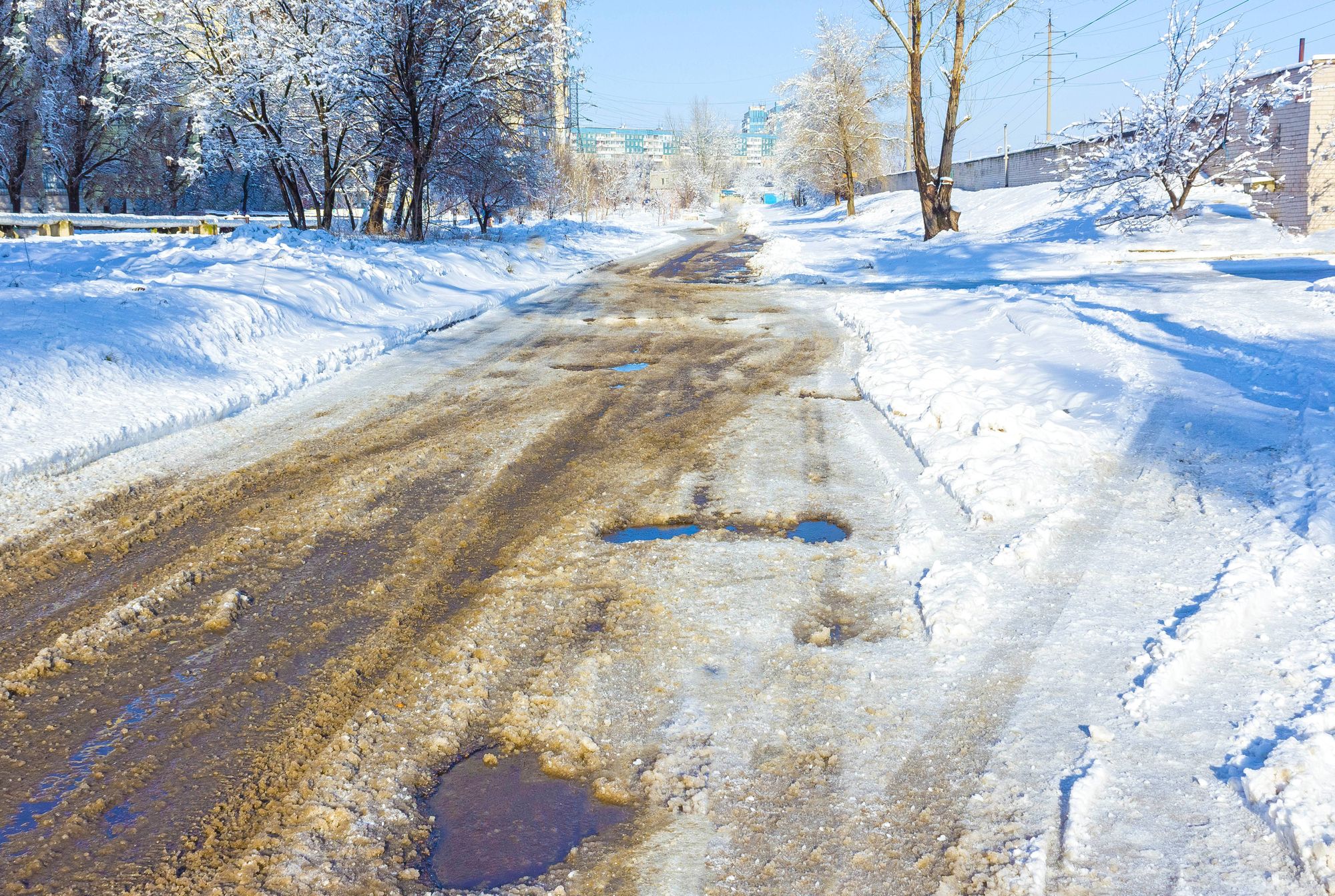The image captures a wintery gravel road winding from the bottom left towards the center of the picture. The road is a mix of brown slush and gravel, interrupted by several small potholes filled with melting snow. Prominent tire tracks are visible, particularly in the center and to the right of the road, emphasizing the muddied, dirty snow streaks. Surrounding the road is a snowy landscape with banks of snow on either side, the right bank being lower than the left. Tall, thin trees dusted with snow frame the background, and a stone wall runs along the right-hand side of the road. In the backdrop, a metal railing and telephone poles rise above the snow-laden scenery, with high power electrical lines stretching into the distance. The sky is a light blue, clear and bright, casting a crisp hue over the scene. In the far background, partially hidden by trees, one can glimpse green and white buildings, adding a hint of human presence to the idyllic winter landscape.